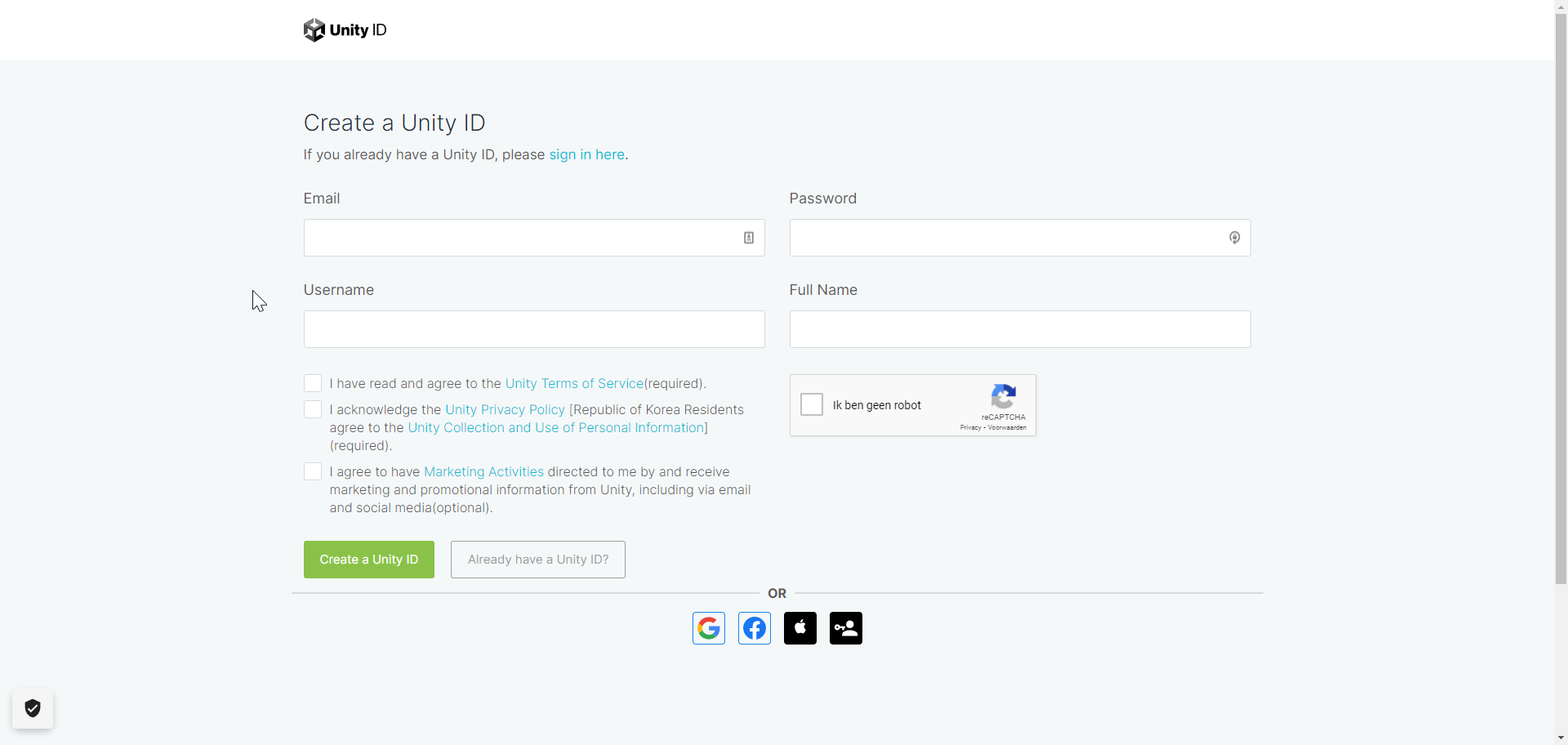This screenshot captures the Unity account creation page, prominently featuring the Unity logo on the top left. The headline reads "Create a Unity ID," accompanied by the instruction, "If you already have a Unity ID, please sign in here," with "sign in here" highlighted in blue as a clickable link.

Below this, the form fields for account creation are displayed, including inputs for email, password, username, and full name. At the bottom of the form are several checkboxes with pertinent agreements:

1. **Mandatory**: "I have read and agreed to the Unity terms of service."
2. **Mandatory**: "I acknowledge the Unity privacy policy."
3. **Mandatory for Republic of Korea residents**: "Republic of Korea residents agree to the Unity collection and use of personal information."
4. **Optional**: "I agree to have marketing activities directed to me by and receive marketing and promotional information from Unity, including via email and social media."

Beneath these checkboxes are two buttons: a green button labeled "Create a Unity ID," and a white button labeled, "I already have a Unity ID?" 

At the bottom of the form, there is a captcha to verify the user is not a robot. Below this, the page offers additional sign-up/in options through Google, Facebook, Apple, or Microsoft accounts, each represented by their respective icons.

In the bottom left corner, there is a security badge icon featuring a checkmark and an armor graphic, indicating some form of verified security feature. This comprehensive layout ensures clarity for users looking to create or sign in to a Unity account.